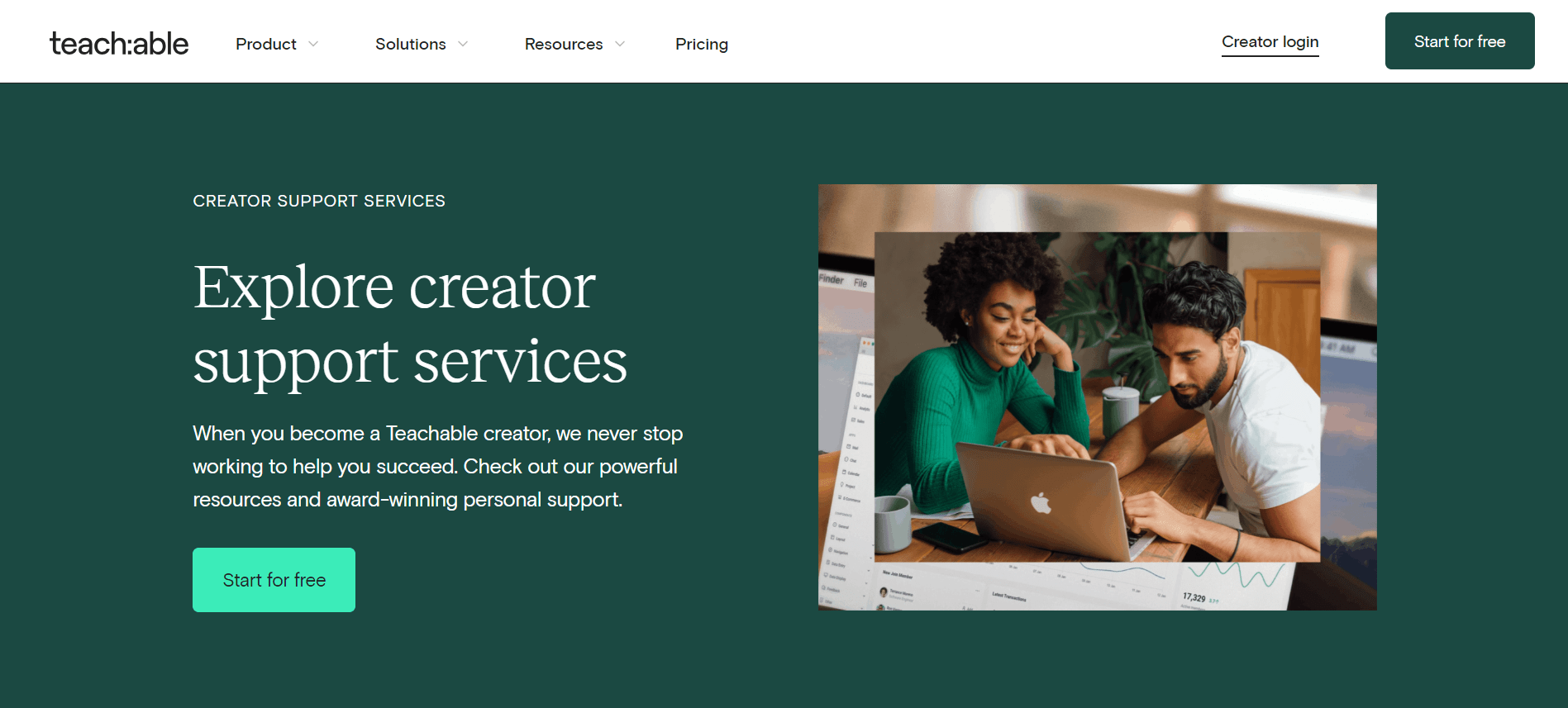The web page for Teachable prominently features the Teachable logo in the top left corner, with the word "TEACH" followed by a colon and "ABLE," spelled out as A-B-L-E. Adjacent to the logo, the menu options include "Product," "Solutions," and "Resources," each with dropdown functionalities, and a "Pricing" option without a dropdown. Next to these menu options, there is a "Creator Login" link, underlined for emphasis. 

Central to the page is a noticeable green button labeled "Start for Free" in white text. The main section features a large green rectangle with the words "Creator Support Services" in bold, white font. Immediately below, the text "Explore Creator Support Services" is prominently displayed. Further down, a smaller text reads, "When you become a Teachable creator, we never stop working to help you succeed. Check out our powerful resources and award-winning personal support." Beneath this, a lighter green button with black text also says "Start for Free."

To the right of this text, there is an image depicting an African-American woman and a white male sitting across from each other at a wooden table, working collaboratively on a MacBook. The woman, seated on the left, wears a green turtleneck, while the man on the right wears a white t-shirt and a bracelet on his left arm. A coffee cup is placed next to the woman. 

In the background of this image, another picture shows a computer screen displaying charts and line graphs, with an indiscernible menu on the left. The farthest background seems to depict the exterior view of a house or an apartment, hinting at a comfortable, home-like setting.